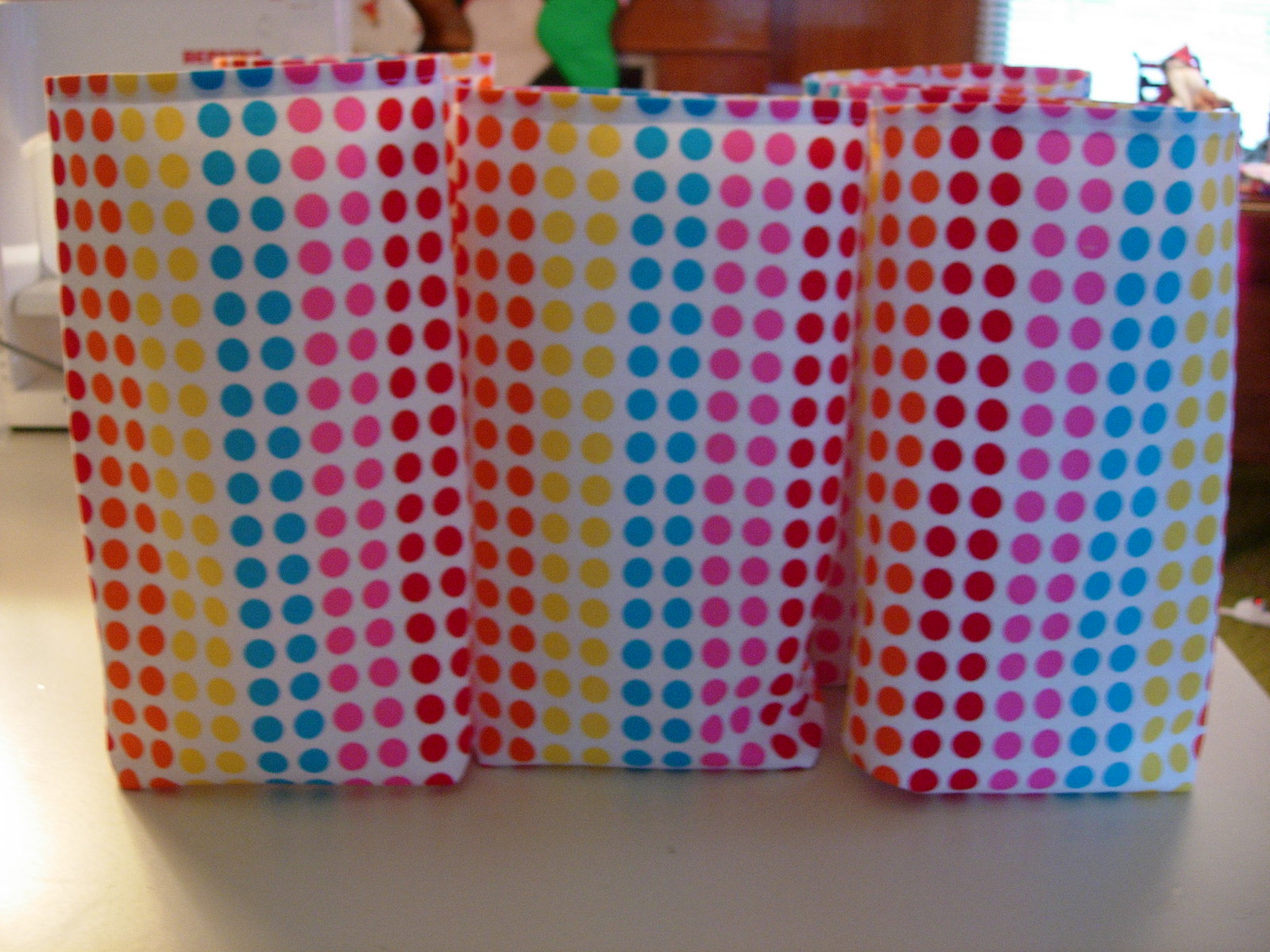The image depicts three large gift bags with polka dot designs on a gray Formica table, positioned in the foreground. Each bag features vertical rows of polka dots in the following sequence: orange, yellow, blue, pink, and red on a white background, repeating around the bags. In the somewhat blurred background, there's an ambiguous indoor setting with hints of home decor, potentially Christmas stockings. A sunlit window with open blinds is visible in the upper right corner, further illuminating the scene. Although there's a suggestion of an additional bag behind the main three, the focus remains on these colorful, upright bags, open at the top and ready for gifting.